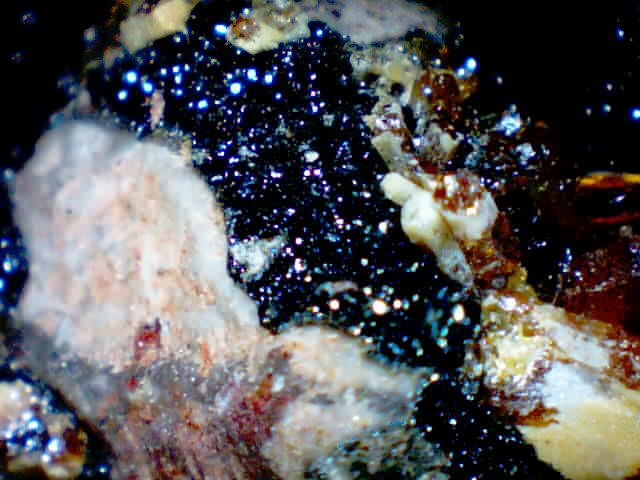This photograph appears to capture a close-up view of a rock or mineral specimen, possibly taken underwater or in a low-light environment given the black backdrop. The specimen features a jagged, irregular shape, with no clear symmetry. It is adorned with a diverse array of colors and textures, making it both sparkly and visually complex. Dominating the center are speckles and flecks of blue and purple, which shimmer and give the impression of lights shining on it. Towards the left side, there are white, translucent jellyfish-like structures accented with hints of red and blue. The right-hand side of the image showcases more distinct yellow and red-colored areas, resembling jellyfish. The upper corners of the photo fade into black, adding a sense of depth, while the bottom left corner reveals more white and blue, lending a frosty, snow-like quality. The entire specimen appears encrusted with various minerals, possibly including elements of brown and golden hues, creating a vibrant and multifaceted appearance.